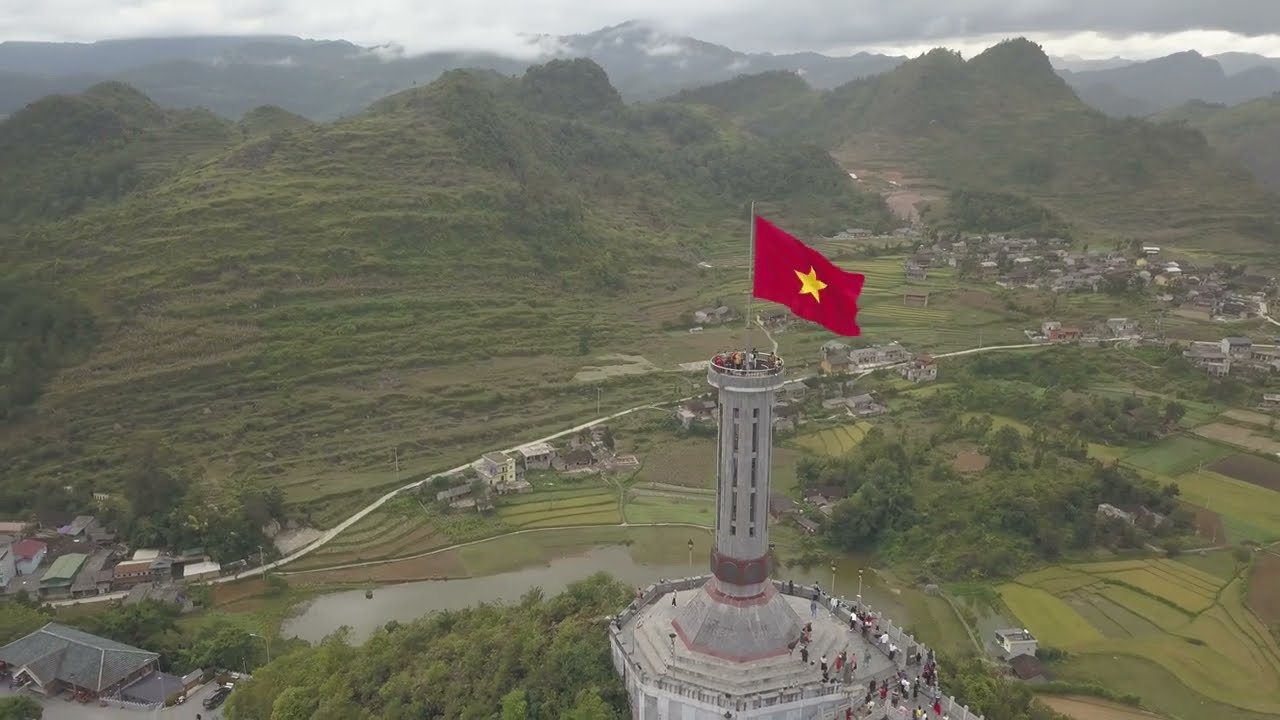The image is an expansive, overhead shot of a picturesque landscape, dominated by a prominent monument at its forefront. At its center, a towering concrete structure rises from a hilltop, characterized by a cylindrical tower perched on a conical or octagonal base, complete with steps and windows leading up to a viewpoint balcony. This viewpoint hosts a red flag adorned with a yellow star, indicating its significance.

Surrounding the monument, a mix of lush farmland and residential areas spread out. The farmland, consisting of alternating shades of green, is interspersed with rice paddies and traditional East Asian buildings, creating a harmonious balance with the natural environment. The residential structures appear more concentrated off to the right and are connected by meandering roads.

Behind this vibrant foreground, a green mountain range occupies the top half of the image, with its uneven, mostly triangular peaks. These green mountains are backed by a darker gray silhouette of another range, enveloped by a bright gray sky filled with white clouds. The cloud line subtly intertwines with the peaks, adding depth and dimension to the composition.

The monument acts as a focal point, bustling with activity as people ascend towards the flag-topped viewpoint and congregate around the base, which is encircled by a small water feature. This dynamic scene, set against the expansive greenery and dramatic mountain backdrop, offers a rich, detailed portrayal of both natural beauty and cultural heritage.